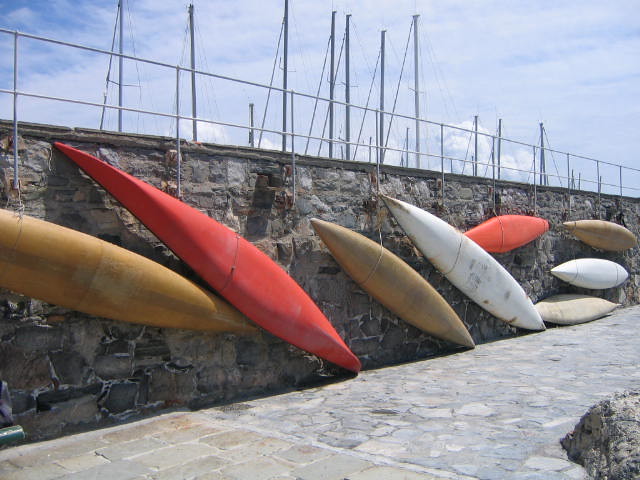A vibrant image showcases a collection of kayaks hung on a large stone wall, contrasted against a backdrop of tall masts from sailboats docked in a marina on the other side. The kayaks, arranged at various angles, feature a palette of colors including bright orange, vivid red, earthy brown, and creamy white. On the right side of the wall, kayaks are hung horizontally, unlike the diagonal arrangement seen elsewhere. The setting includes a concrete and stone cobblestone walkway in the foreground, with a piece of contrasting lava rock visible in the bottom right corner. A metal fence tops the wall, and the entire scene is bathed in sunshine under a clear blue sky.